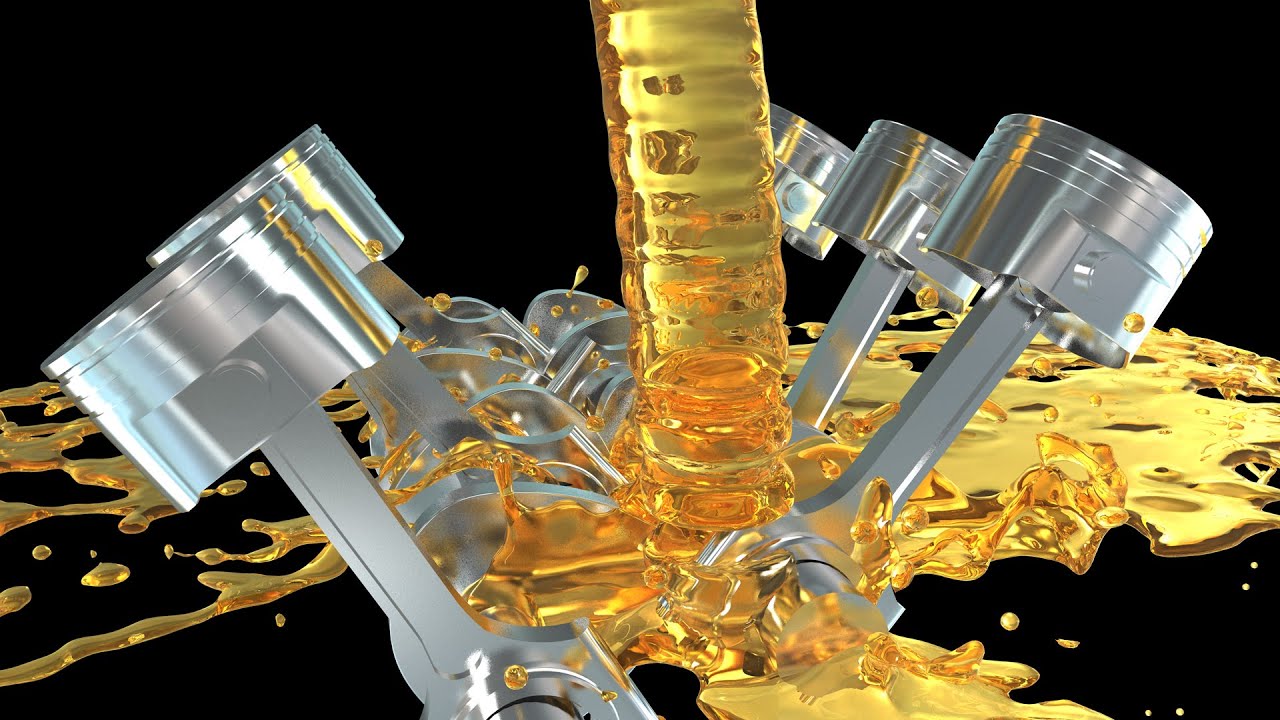This 3D-rendered image depicts a detailed scene of six shiny, steel pistons emerging from what appears to be an engine block. The pistons, three on each side, are arranged in a V-shape formation, standing upright with connecting rods and round tops. A golden, translucent liquid, resembling motor oil or honey, cascades down from a tube at the center of the image, splashing onto the pistons below. This liquid then spreads and splatters across the metallic surfaces, creating a dynamic contrast against the stark black background. Small splashes of the gold liquid decorate the pistons, emphasizing the fluid motion and impact. The overall scene combines realistic textures and lighting to create a striking visual of mechanical components interacting with the flowing liquid.